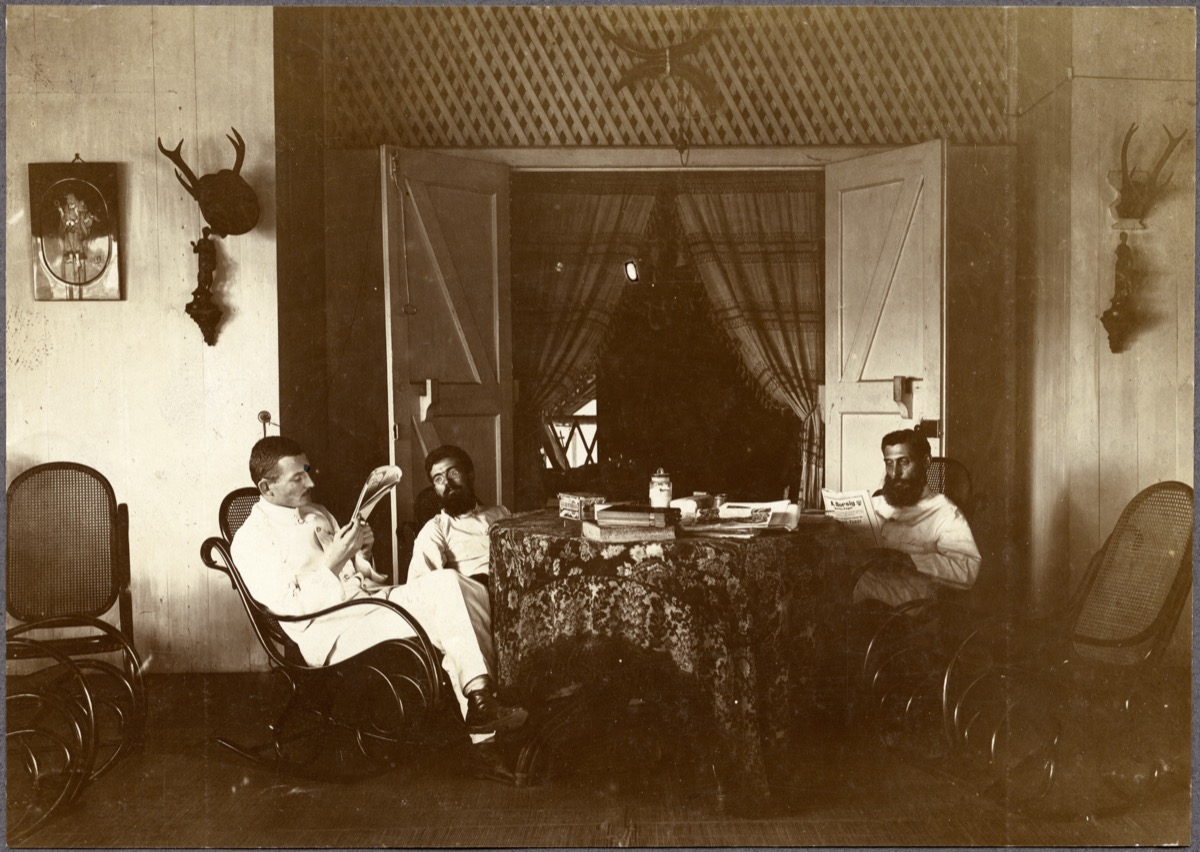This sepia-toned, black-and-white photograph captures a scene of three white men seated around a tall, round table covered with a floral tablecloth that drapes to the floor. Two of the men, characterized by their heavy, bushy beards and dark hair, are leaning back in their wicker-backed rocking chairs, while the third man, dressed in a white suit and black leather shoes, sits in an old-style wicker rocking chair reading a newspaper. This third individual, either clean-shaven or with a mustache, has short-cropped hair, different from the slightly longer hair of his companions. 

The setting appears to be a communal or recovery area, with walls made of wooden boards. On the right side of the room, there is a mounted deer head and a small statue, possibly an oil lamp featuring a woman's figure, which is mirrored on the left side. Above the wide-open French barn-style doors, flanked by plaid curtains, is a horizontal wooden lattice design. The doors themselves are topped with a pair of horns arranged in a mirrored fashion. The room has a somewhat dark ambiance, and various indistinct items, possibly books or boxes and an object resembling a sugar or creamer jar, are spread across the table.